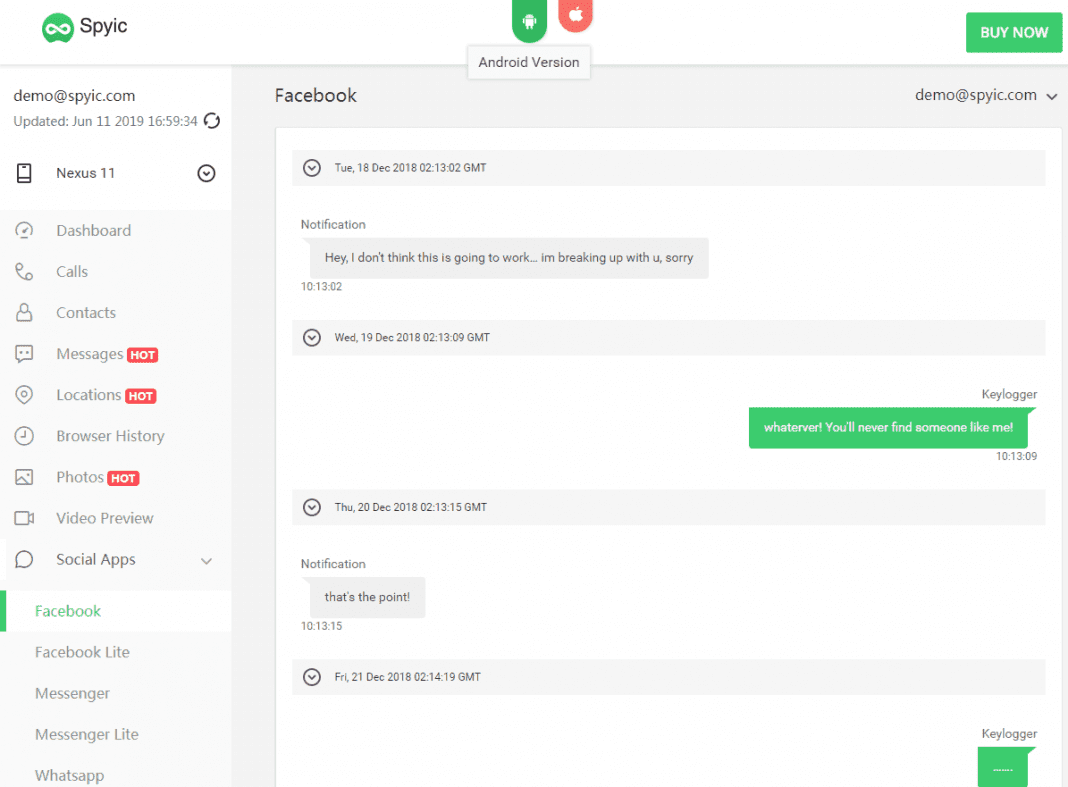**Detailed Caption:**

The image displays the web interface of SpyIC, an online monitoring tool, accessible through the demo at spyic.com. It reflects an updated layout as of June 11, 2019, featuring a comprehensive dashboard. The sidebar menu includes tabs for Calls, Contacts, Messages, Locations, Browser History, Photos, Video Preview, and Social Apps such as Facebook, Facebook Lite, Messenger, Messenger Lite, and WhatsApp.

Key details highlighted in the image include:

- **Date and Time**: Notifications from the tool are timestamped, with one significant message displayed as "Tuesday, 18th of December, 2019, 2:13 GMT" under O2 network. The message reads: "Hey, I don't think this is going to work, I'm breaking up with you, sorry."

- **Keylogger Section**: Another timestamp "Wednesday, 19th December, 2018, 2:13 GMT" shows an entry from the keylogger capturing a message, "whatever, you'll never find someone like me." This message continues with a second entry stating, "That's the point, keylogger...", suggesting a dialogue captured by the tool.

- **Visual Elements**: The interface uses distinct color codes for various elements like green, red, and whites, presumably to denote different states or types of information (e.g., notifications, alerts, and logs).

The dashboard’s organized structure and color schemes help users easily navigate through collected data, offering a snapshot into digital interactions and activities.